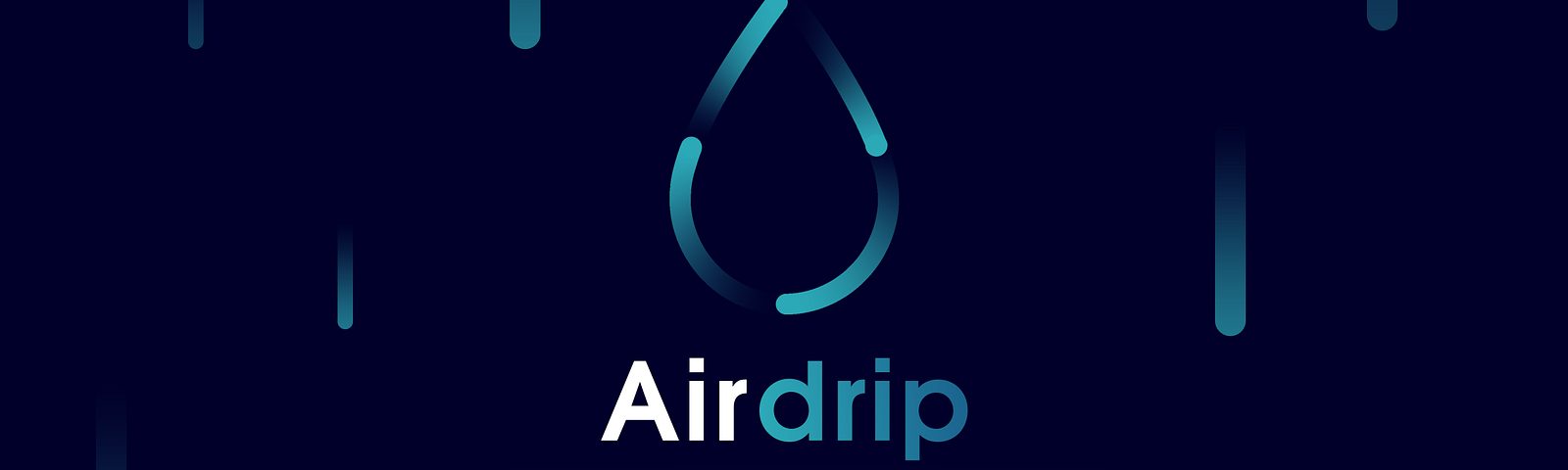The image features a horizontal strip with a dark navy blue background. Light turquoise droplets are falling from the top of the strip, creating a cascading effect. In the center of the image, some of these droplets coalesce into the shape of a larger water droplet. Directly beneath this central droplet is the word "AIR DRIP" — the word "AIR" is in uppercase white font, while "DRIP" is in the same turquoise color as the droplets, ensuring a consistent theme throughout. This image likely serves as a logo, possibly for a company named Air Drip, with an emphasis on the interplay of water imagery and typography.